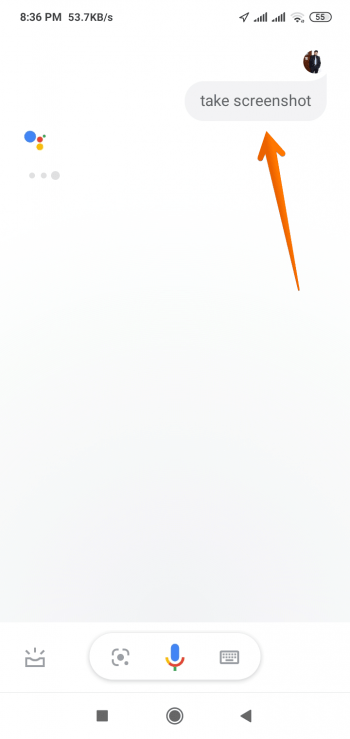The image is a vertically oriented rectangle resembling the interface of a smartphone. At the top of the screen, there's text displaying "8:36 PM" followed by "53.7 KB/s" in black. On the right side, there's an arrow pointing to the upper right, along with two fully-filled cell phone service bars and a faint Wi-Fi signal icon. Additionally, a circled number "55" is present.

Below this, there's a circular avatar icon representing a person, followed by a dialogue box that reads "Take screenshot." A large orange arrow is directed upwards towards this dialogue box. The background in this section is light gray.

At the bottom of the screen, there's an elongated rectangular area containing three icons: a square-like symbol, a microphone, and a keyboard icon. Beneath this is a thin gray line with three more symbols underneath: a square, a circle, and a triangle pointing to the left.